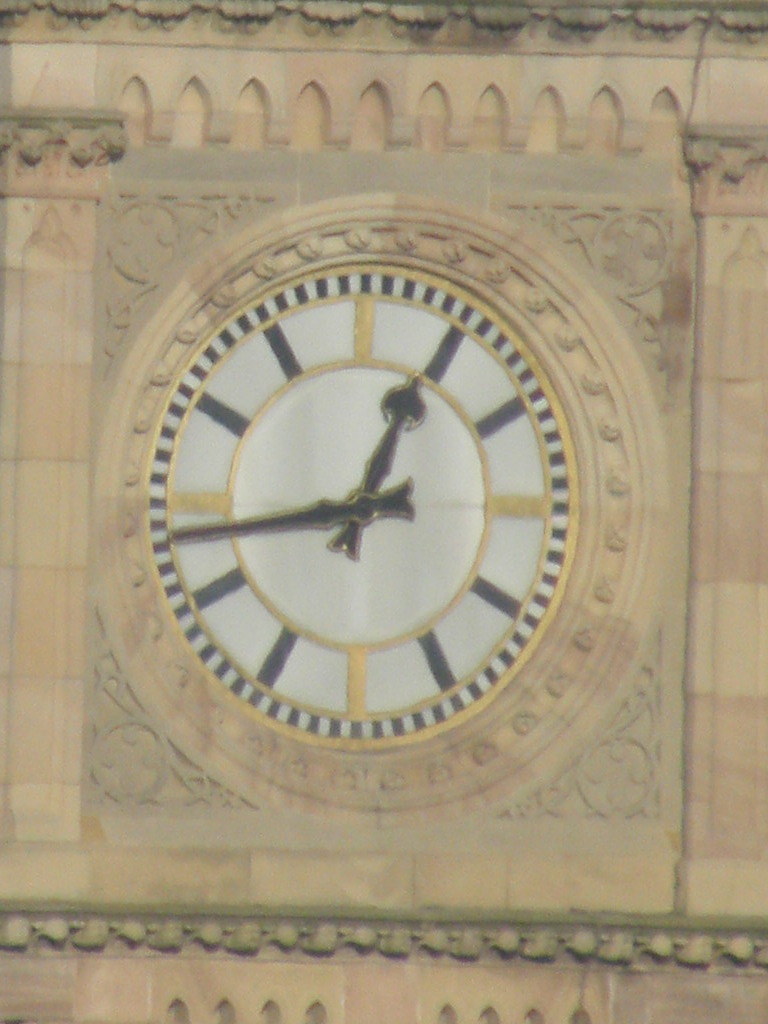This image features a beautifully chiseled clock embedded into a stone building facade. The clock face is stark white, contrasting sharply with its black hands. The minute hand is pointing slightly before the equivalent of the nine o'clock position, while the hour hand is nearing the one o'clock mark, indicating the time is approximately sixteen minutes to one. The clock face itself is devoid of any numerals. Surrounding the clock are intricate stone carvings that add an element of grandeur and meticulous craftsmanship to the structure. Directly above the clock, a series of small, sculpted arches enhance the architectural elegance of the overall design.